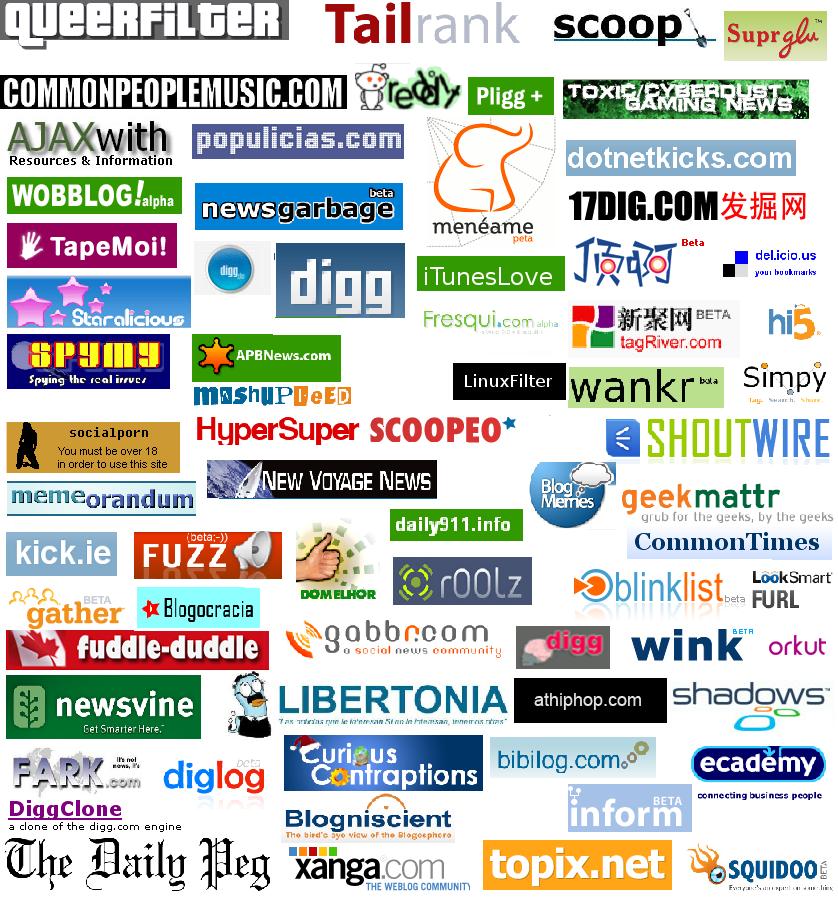The image displays a grid of colorful bumper stickers or logos for a variety of old internet websites and services. Arranged in a 4 by 16 format, the stickers feature names like "Queer Filter," "Tail Rank," "Scoop," "Superglue," "CommonPeopleMusic.com," "Reddit," "Plig," "Toxic," "Cyber Dust," "Gaming News," and "Ajax with Resources and Information." Each sticker stands out with different colors including green, red, blue, yellow, orange, purple, and pink, set against a white background. The stickers and text vary in shape, with some being standalone text while others are rectangular. The array also includes names such as "Populicious.com," "Manyammy.netkix.com," "Wobblog Alpha," "News Garbage Beta," "iTunes Love," "17dig.com," "Tape Moi," and "Staralicious," capturing a nostalgic snapshot of early internet culture with a vast diversity of titles and vibrant hues.